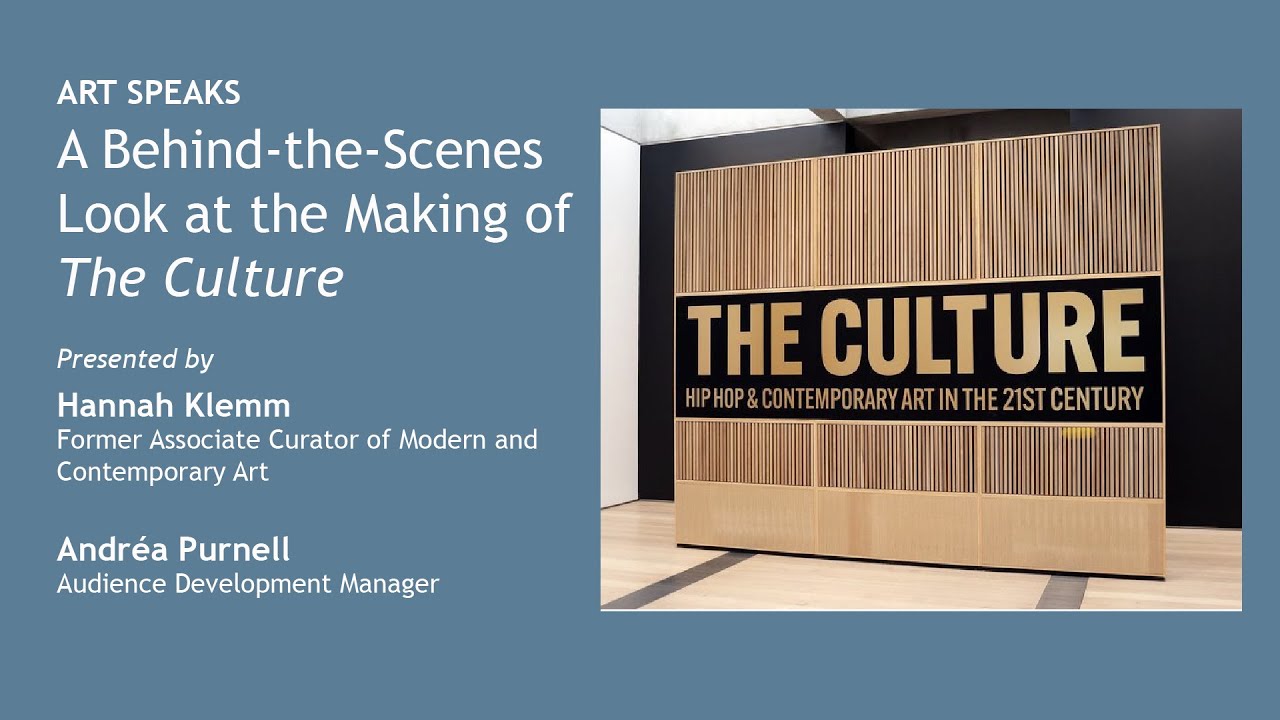The image features a promotional slide, reminiscent of a website or PowerPoint presentation, with a light blue background and white text that reads "ART SPEAKS" in all capital letters. Below it, in smaller text, it states "A behind-the-scenes look at the making of The Culture, presented by Hannah Clem, former Associate Curator of Modern and Contemporary Art, and Andrea Purnell, Audience Development Manager." On the right side of the slide, there is a photograph of a large display sign positioned inside a building. The sign has a brown background with thin black stripes and features a prominent black box bordered in gold. Inside the box, in large gold capital letters, it reads "THE CULTURE," with "Hip Hop and Contemporary Art in the 21st Century" written beneath it in smaller capital letters. The display appears to stand approximately six feet tall and ten feet wide, placed on a wooden floor, with overhead lighting and a white ceiling visible in the background. This detailed and visually striking slide effectively markets an insightful lecture on contemporary culture and art.